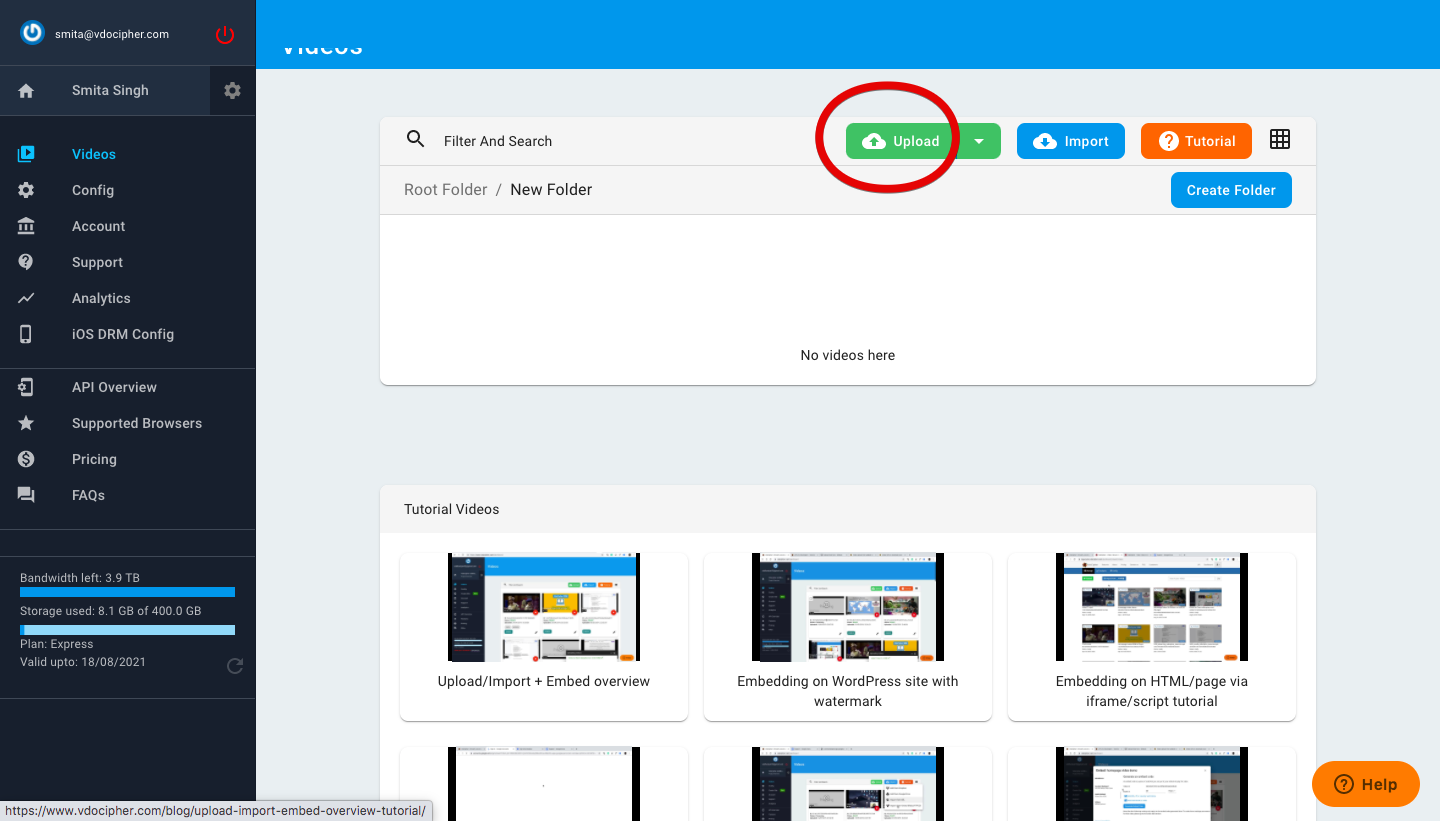This screenshot captures the admin dashboard of a WordPress site, featuring a clean and organized layout. Dominating the left side is a dark gray sidebar that frames the central workspace.

At the very top of the sidebar, an email address associated with wordpress.com is prominently displayed, followed by a red power button icon. Just below, the username "smitesync" is positioned between a home icon on the left and a settings gear icon on the right, conveying administrative privileges.

The sidebar itself is neatly divided into sections. The first section contains six navigation buttons: "Videos," "Config," "Account Support," "Analytics," "iOS DRM Config," each accompanied by a relevant icon on their left, providing quick access to core functionalities. A dividing line separates these from the next set of options.

The second section lists four more items: "API Overview," "Supported Browsers," "Pricing," and "FAQs," each also featuring an icon on the left, facilitating easy navigation for users seeking specific information or settings. The overall design is intuitive, with clear visual cues that guide users effortlessly through the dashboard's various features.